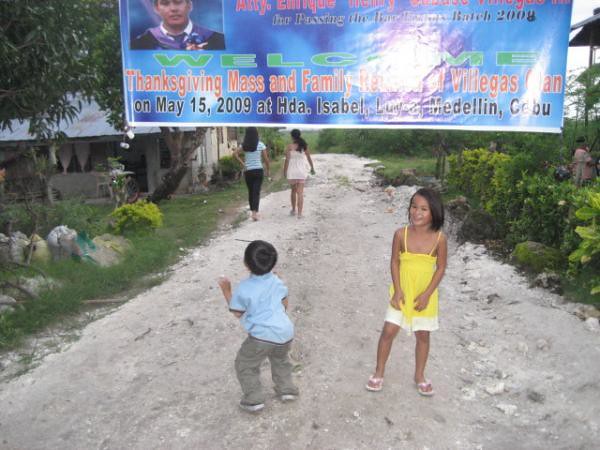In the image, two young children, a boy and a girl, are standing outside on a dirt and rock pathway, surrounded by greenery. The pathway seems to be a light gray or whitish color, with green bushes on the right and green grass on the left, along with some gray rocks and trees with lush green leaves. A house with a gray sidewall and a shiny, flat steel roof is partially visible in the background. The children are positioned under a banner that reads "Welcome Thanksgiving Mass and Family" with additional text indicating the event is on May 15, 2009 at HDA Isabel in Medellin. The blue banner with green and orange text is slightly obscured by sun flare, making some details hard to read. The girl, who has dark brown skin, black hair, and is possibly South Asian, is wearing a yellow dress with white flip-flops and is smiling at the camera. The boy, with short black hair, is wearing a light blue shirt, dark gray pants, and dark shoes with white soles, and has his back turned, looking up at the banner. Additionally, two young women can be seen walking away in the background.